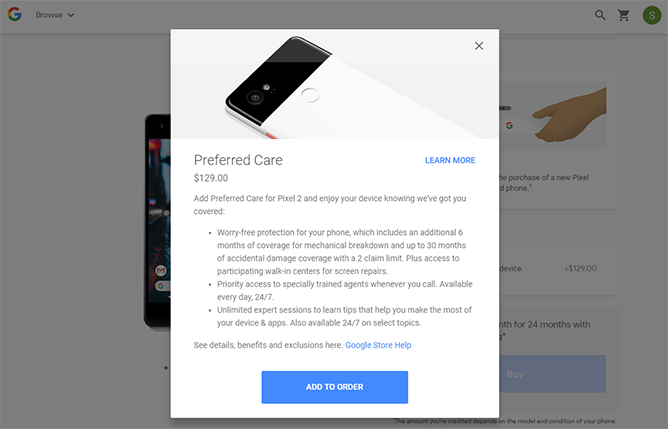This image is a screenshot of a Google Store page. At the top of the page, the distinct Google icon featuring the colorful "G" is visible, along with a "Browse" option accompanied by a drop-down arrow. To the right of these features, there is an "S" icon indicating a user who is signed in, a shopping cart icon, and a magnifying glass icon for search functionality.

The screenshot focuses on a product page for "Preferred Care." Dominating the center of the screen is a pop-up box detailing the Preferred Care service offered for the Pixel 2. The service is priced at $129. The description states: "Add Preferred Care for Pixel 2 and enjoy your device knowing we've got you covered." The product offers several features, including coverage for damage lasting up to 30 months, priority access to trained agents available 24/7, and unlimited expert sessions for tips, also accessible 24/7.